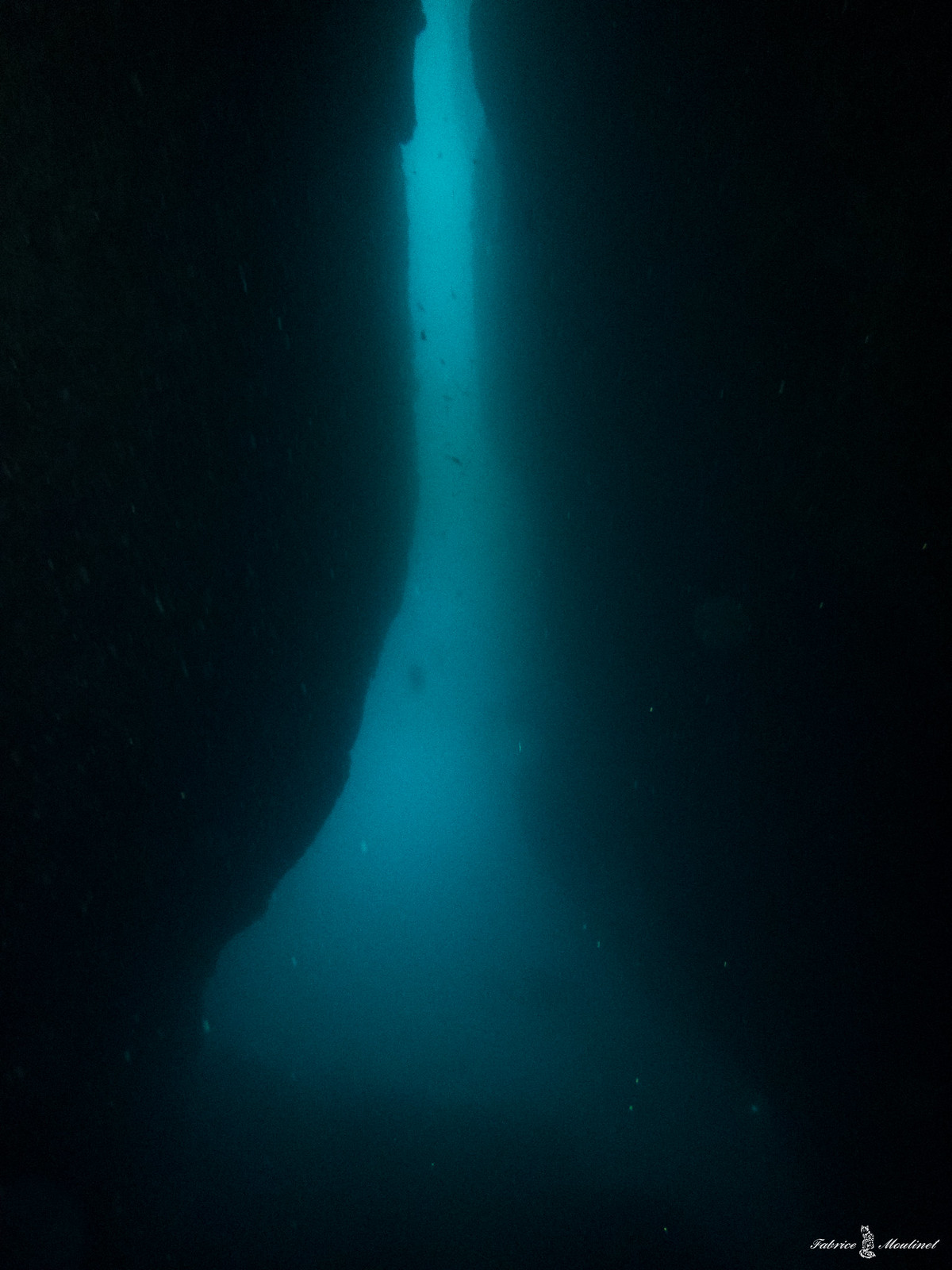This underwater image captures a murky, low-lit scene within a crevice or cavern flanked by two massive rock faces. The water appears cloudy, giving the scene a blurry quality. In the center of the image, a thin strip of lighter blue water is visible, suggesting deeper penetration of light, which contrasts sharply with the darker, more obscure hues dominating the edges, especially the upper left and right corners. Throughout this central strip, a variety of objects—likely fish—are seen swimming, with some appearing larger and others smaller. Additionally, there are small, floating flecks that glisten when catching the light, juxtaposed against darker, shadowy particles, possibly debris or rocks. Towards the bottom right and left corners, a barely readable white text logo or label is present, further adding to the enigmatic underwater tableau.